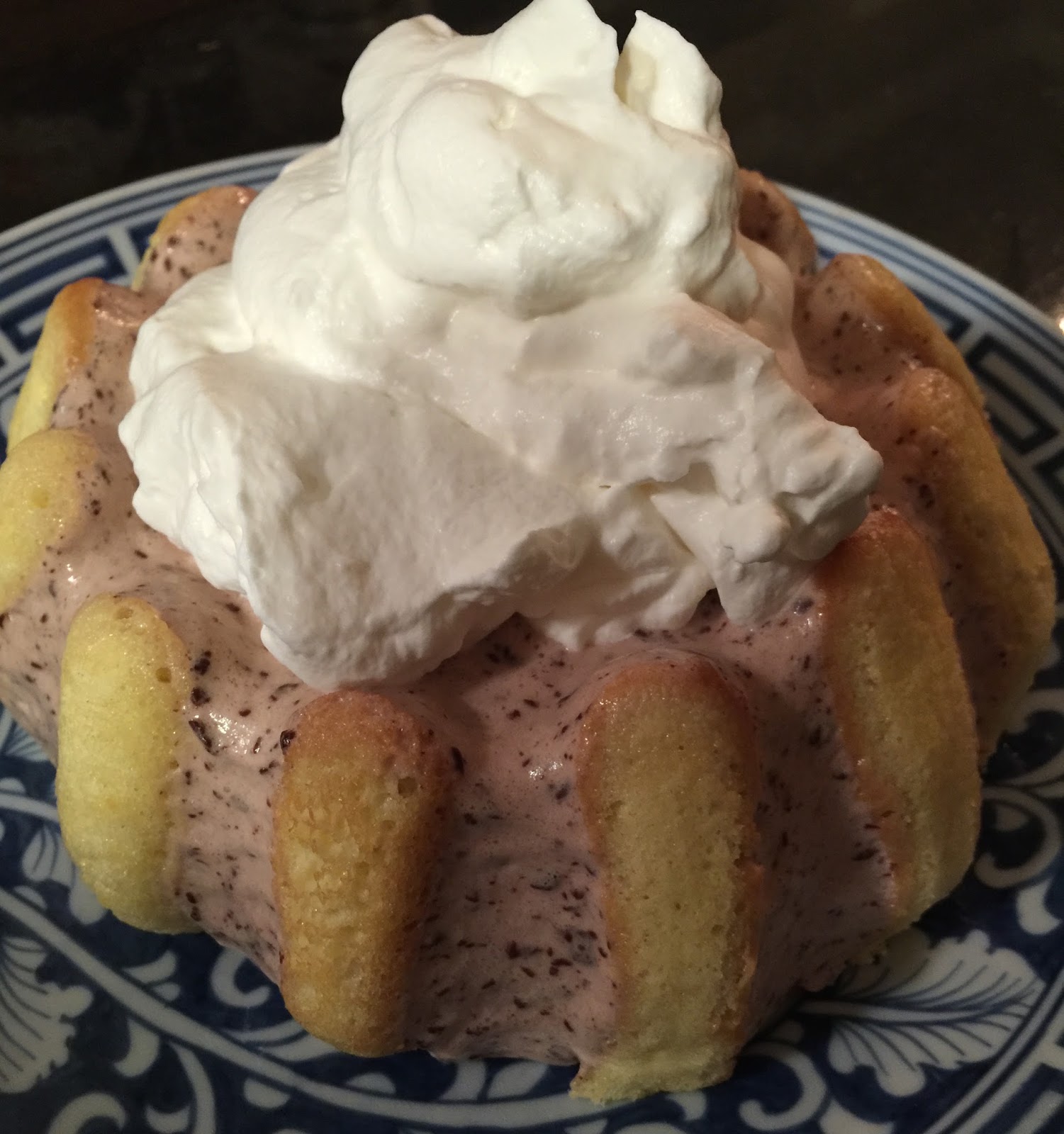This close-up image features a delectable Bundt cake, presented on a vintage blue plate adorned with intricate white floral and leaf designs. The cake itself is a light vanilla sponge, its elegant shape formed by the distinct ridges of the Bundt pan. At its center, an inviting layer of brownish icing speckled with dark flecks enhances its appeal. Topping this, a generous dollop of slightly melty whipped cream, the kind dispensed from a can, adds a touch of indulgence. The background sets a contrasting tone with its dark, blackish-brown color, further highlighting the dessert's exquisite presentation. This dessert, with its thoughtful combination of flavors and textures, epitomizes culinary elegance and readiness to be savored.